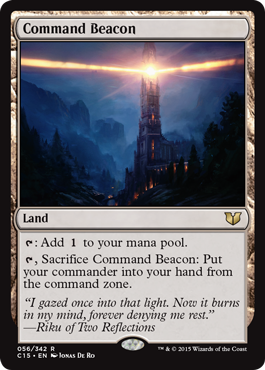The image depicts a card titled "Command Beacon," featuring prominent dark black edges. At the center of the card is a round, silver emblem with a black core. The scene is set at nighttime, with a dark atmosphere enhanced by occasional lit windows in the background. Rising prominently is the Command Beacon tower, its apex emitting brilliant, daylight-like rays shooting outward to the left and right, piercing through the surrounding clouds. 

At the bottom left corner, stone walls frame the scene, leading to dark, obscured trees at the very edges. Positioned below the artwork on the left is the designation "Land," while the right features a small gold shield. The text below reads: "Add one mana of any color to your mana pool," followed by, "Sacrifice Command Beacon: Put your commander into your hand from the command zone." An evocative flavor text at the bottom states, "I gaze once into that light, now it burns so in mine, forever adoring you as we go to reflections."